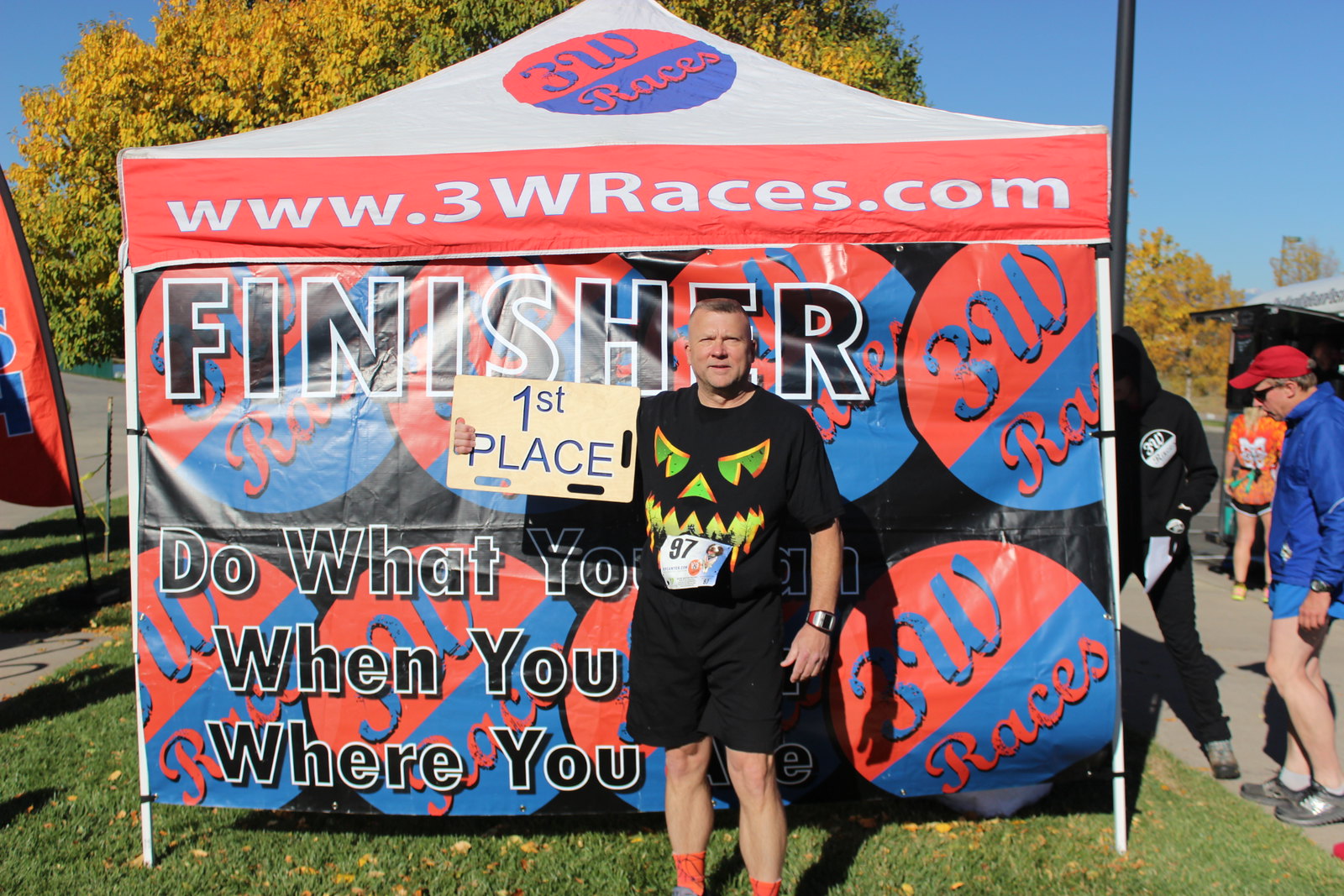In this vibrant and detailed image captured at a race event in early autumn, a man stands proudly in front of a tent adorned with colorful graphics and logos from 3W Races. His black t-shirt features an abstract jack-o'-lantern face with green eyes and a green mouth, mirroring the Halloween theme. He wears black shorts, a red watch on his left wrist, and has the number 97 pinned to his shirt. Holding a "First Place" sign high, he gazes confidently into the camera. The backdrop tent reads "Finisher" in bold letters and carries the motivational slogan "Do what you want, where you want, when you want," with the event website www.3wraces.com prominently displayed. Surrounding the tent, the scene includes several other figures, such as a man in a black hoodie, another racer with a number on her jersey, and a man in a blue hoodie. The setting is filled with green grass dotted with brown leaves and orange-hued trees, under a clear blue sky, perfectly capturing the crisp, sunny, fall day.